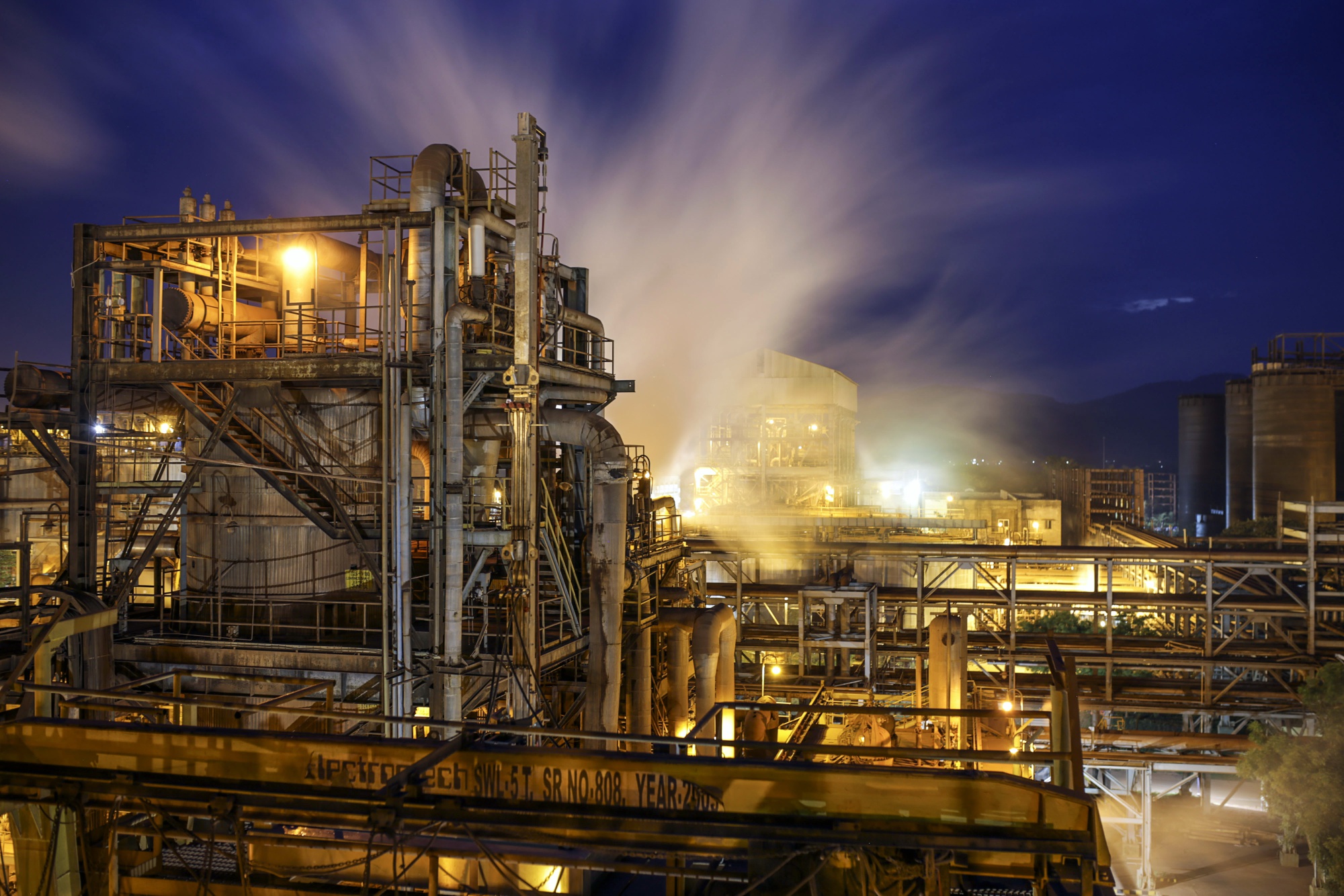This nighttime photograph captures a sprawling industrial complex set against a dark blue sky strewn with fog and billowing smoke. Dominating the scene are several large cylindrical silos, both metal and concrete, prominently situated with a massive array of interconnected pipes, steel beams, and staircases weaving throughout the structure. The facility is drenched in an eerie yellow light, illuminating various platforms and walkways, as if highlighting the vastness and complexity of the workspace. Clouds of smoke or gas emanate from the center of the factory, lending a foreboding atmosphere suggestive of active chemical or industrial processes. In the distance, the silhouette of mountains is visible, accentuating the factory's remote location. Text reading "fifth SWL5TSR number 808 year 2000" is faintly visible on a guardrail, further emphasizing the factory's mysterious and archaic allure.